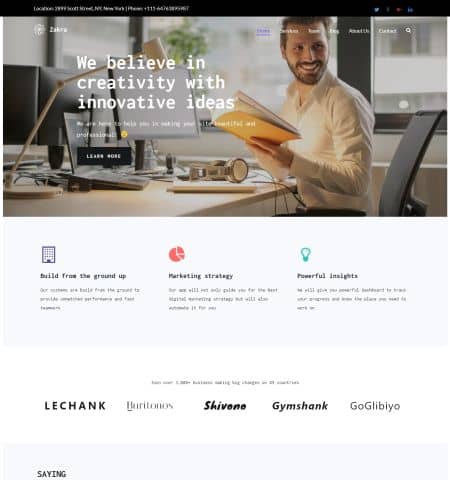The image depicts a webpage with various elements centered around a business theme. At the top, there is a black bar with white text and several social media icons on the right-hand side. Below this bar, the headline reads, "We believe in creativity with innovative ideas." Some additional, lower-resolution text follows that is difficult to decipher.

In the background, behind the text, there is a photograph of a man seated at a desk. He is a white male with a friendly smile, wearing a white long-sleeve shirt. The setting appears to be a bright room, as natural light streams in through nearby windows. On his desk, he has a notebook open in front of him, along with a computer, a lamp, and a pair of headphones.

Further down the page, there are three distinct sections titled "Build from the Ground Up," "Marketing Strategy," and "Powerful Insights." Following these sections, a few company logos can be seen, including names like LeChank, Bartonio, Chavin, Jim Shank, and GoGliblio.

At the very bottom, there is a partially readable text that repeats itself but is somewhat unclear. It appears this webpage is related to business solutions or office productivity. An icon starting with the letter "Z" is positioned in the upper-left corner, though the full name is not legible. Lastly, a black "Learn More" button with white text is situated somewhere on the page, inviting further exploration.